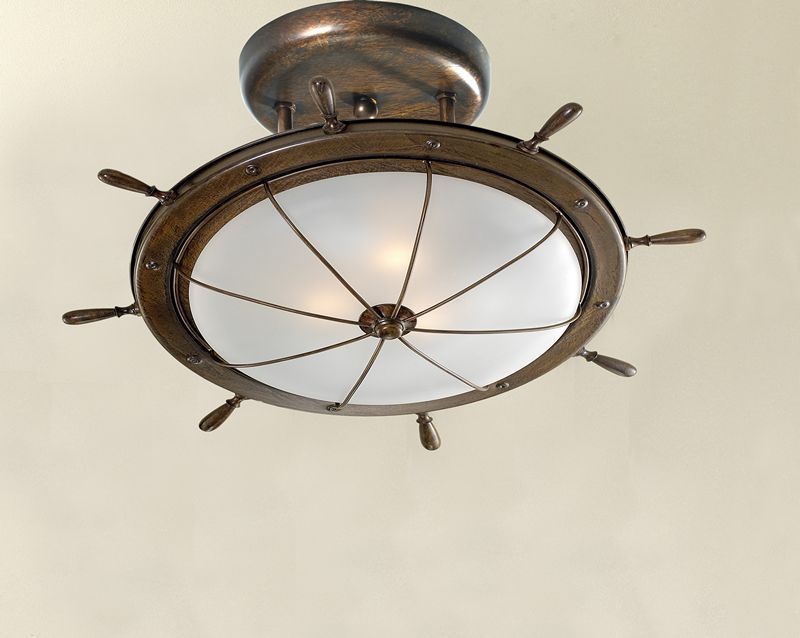This photo showcases a unique, nautical-themed ceiling light fixture designed to resemble a traditional ship's wheel. The light fixture features a bronze metal frame with eight handles, which mimic the spokes of a ship's wheel, encircling a central dome of frosted glass. The frosted glass is distinctively divided into eight segments, adding complexity and visual interest to the design. The fixture is mounted to the ceiling via a small, oval wooden base, giving the illusion of it hanging. The ceiling itself appears to be white, contrasting nicely with the dark brown wood and bronze elements of the fixture. The background behind the fixture is a light gray, further enhancing the overall aesthetic.